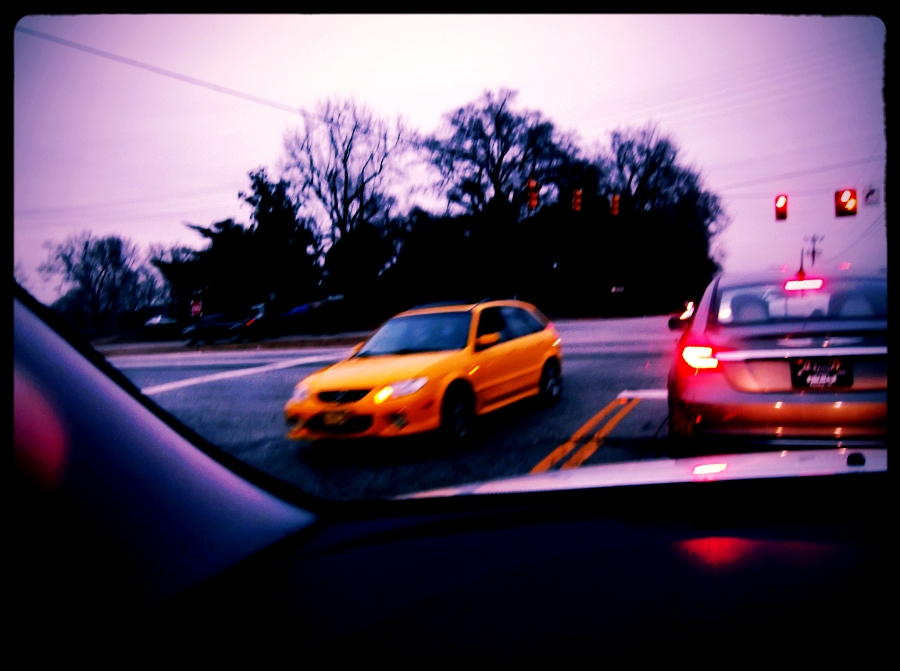The photograph is taken from the dashboard of a black-interior vehicle with a white frame, capturing a daytime scene outside. Directly ahead, a silver car with illuminated brake lights is partially visible off the right side of the frame, stopped at an intersection governed by five traffic lights showing red. To the left, an oncoming yellow sedan with its left turn signal flashing approaches the intersection. Overhead, electrical wires hold up the traffic lights, and a barely discernible sign with a black right-pointing arrow adds to the roadside details. The setting includes a small wooded area with varying leaf density on the trees. The scene has a slightly out-of-focus, purplish-violet tint, giving it a Lumography-style effect.